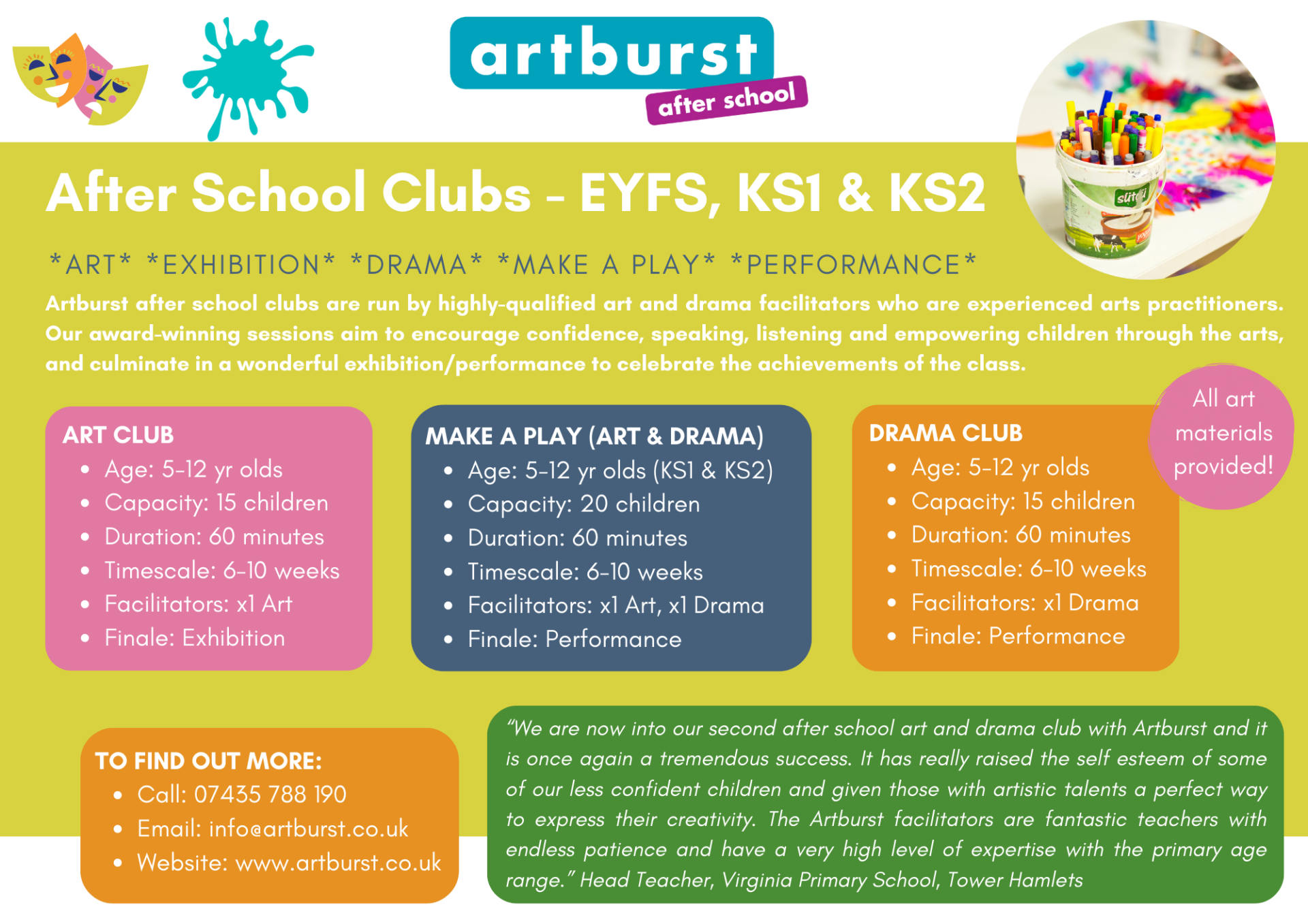The vibrant and detailed poster features a prominent teal rectangle with rounded corners at the top, reading "Art Burst" in white text, followed by a purple rectangle below stating "After School." In the top left corner, there are drama masks – a happy and a sad face – alongside a teal paint splotch. On the top right, a small circle encloses an image of a bucket of crayons. Centered below is a large pale green rectangle containing white text detailing the offerings: "After School, EYFS, KS1, and KS2," along with activities such as "Art Exhibition," "Drama," "Make a Play," and "Performance."

The poster elaborates on the various programs available, including "Art Club," "Drama Club," and "Make-A-Play," each described in colorful rectangles – purple, blue, orange, and green – with additional white text providing specifics about age groups (5-12 years old), session lengths (60 minutes), and durations (6-10 weeks). The green rectangle highlights a testimonial, while a pink triangle on the right middle section emphasizes "All art materials provided."

Highly qualified art and drama facilitators run the sessions, focusing on building confidence, enhancing speaking and listening skills, and empowering children through the arts. The program culminates in an exhibition or performance to celebrate the students' achievements. For more information, contact details, including a website link, are provided.